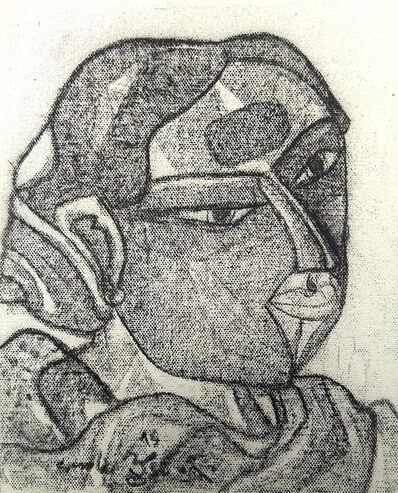The artwork is an abstract black and white depiction of a human face, with the figure turned towards the right. It is crafted on an ivory-colored fabric, causing the lines and details to blend slightly and appear somewhat blurry. The stylized face, reminiscent of hieroglyphic design, is characterized by geometric shapes and divided into distinct sections. The person appears to be a woman, with short hair, a pronounced long nose reaching down to a diamond-shaped mouth, and a noticeable oblong patch on the forehead. Her eyebrows nearly touch each other, contributing to her intense expression. She is adorned with a headpiece or scarf. The piece is rendered from the top of her head to her upper shoulders, pointing towards the bottom right. A faded and hard-to-read signature and the number 19 are located at the bottom left corner. The entire composition is outlined in black and white, set against a white and grey background.